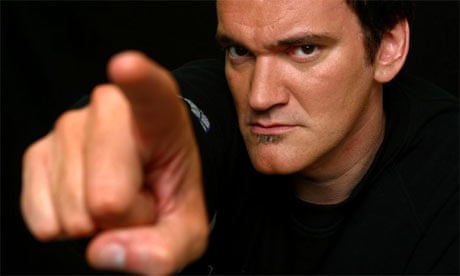The photograph is a close-up of a young Quentin Tarantino, centered from the top to about the middle of the image. His expression is intense, with furrowed brows and an angry look, his mouth firmly shut. He has short black hair and a small patch of hair under his bottom lip, adding to the serious demeanor. His chin is pronounced with a cleft, and his jaw juts out slightly. Tarantino's eyes are dark and piercing. His right hand extends towards the camera, with his finger pointing directly at the viewer. The tip of his finger is blurry due to the close proximity to the lens. The background is completely black, blending seamlessly with his black shirt, making it difficult to distinguish where his clothing ends and the background begins. The dramatic lighting and dark tones emphasize his intense expression and the overall mood of the photograph.